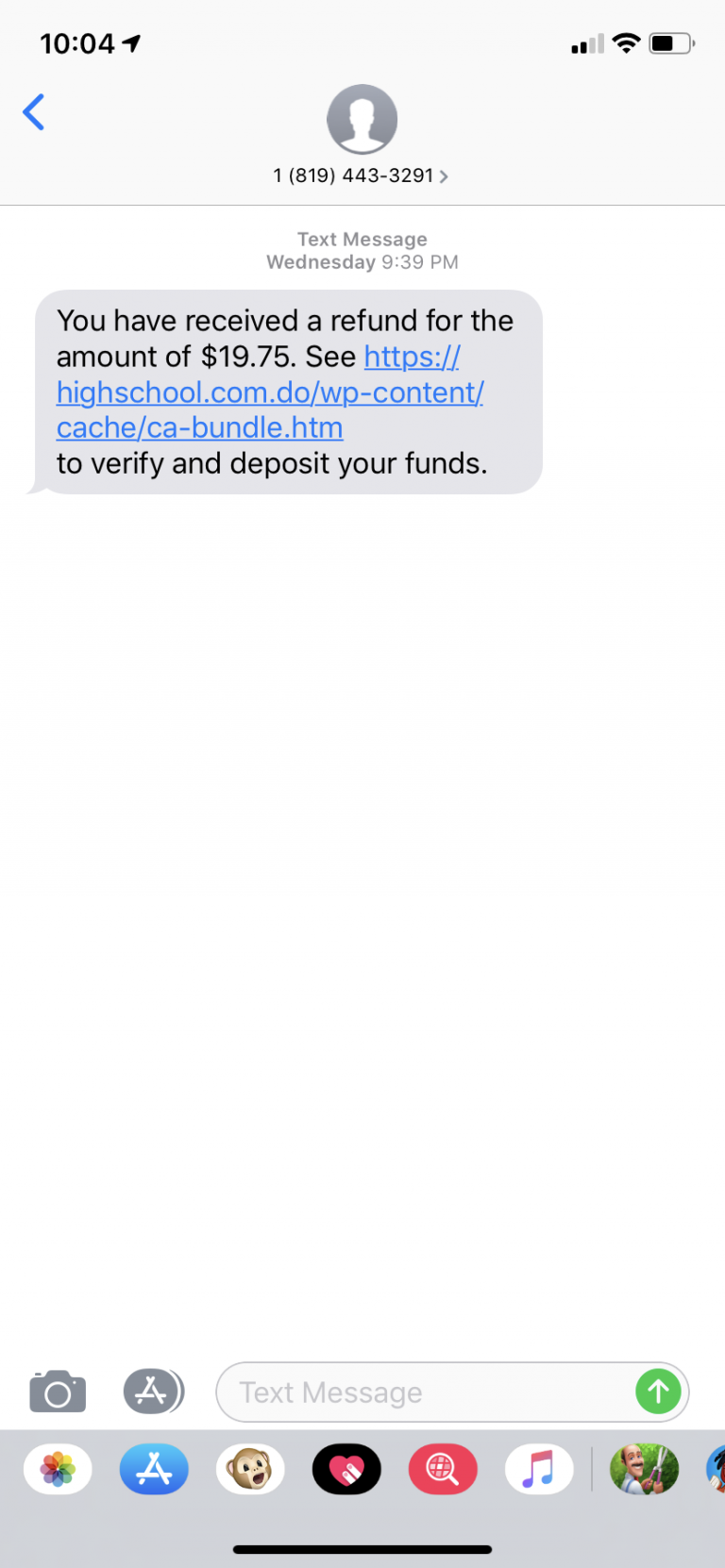This is a screenshot of a mobile phone text message conversation. At the top left corner of the image, the time is displayed as 10:04. To the right of the time, there is a small black arrow pointing slightly to the right. On the top right corner, three icons are visible: a cellular signal bar icon, a WiFi signal icon, and a battery icon showing 50% charge.

Centered at the top of the screen is a silhouette avatar of a person, below which is displayed the contact number "1-819-443-3291." The text message was sent on Wednesday at 9:09 PM and reads: "You have received a refund for the amount of $19.75. See highschool.com. It's a URL to verify and deposit your funds." 

The background of the text message window is white, and the message itself is contained within a light gray speech bubble. At the bottom of the text message window, there is a camera icon, an "A" icon inside a circle, and a text input bar. To the right of the text input bar is an upward-facing arrow inside a green circle, signaling the send button.